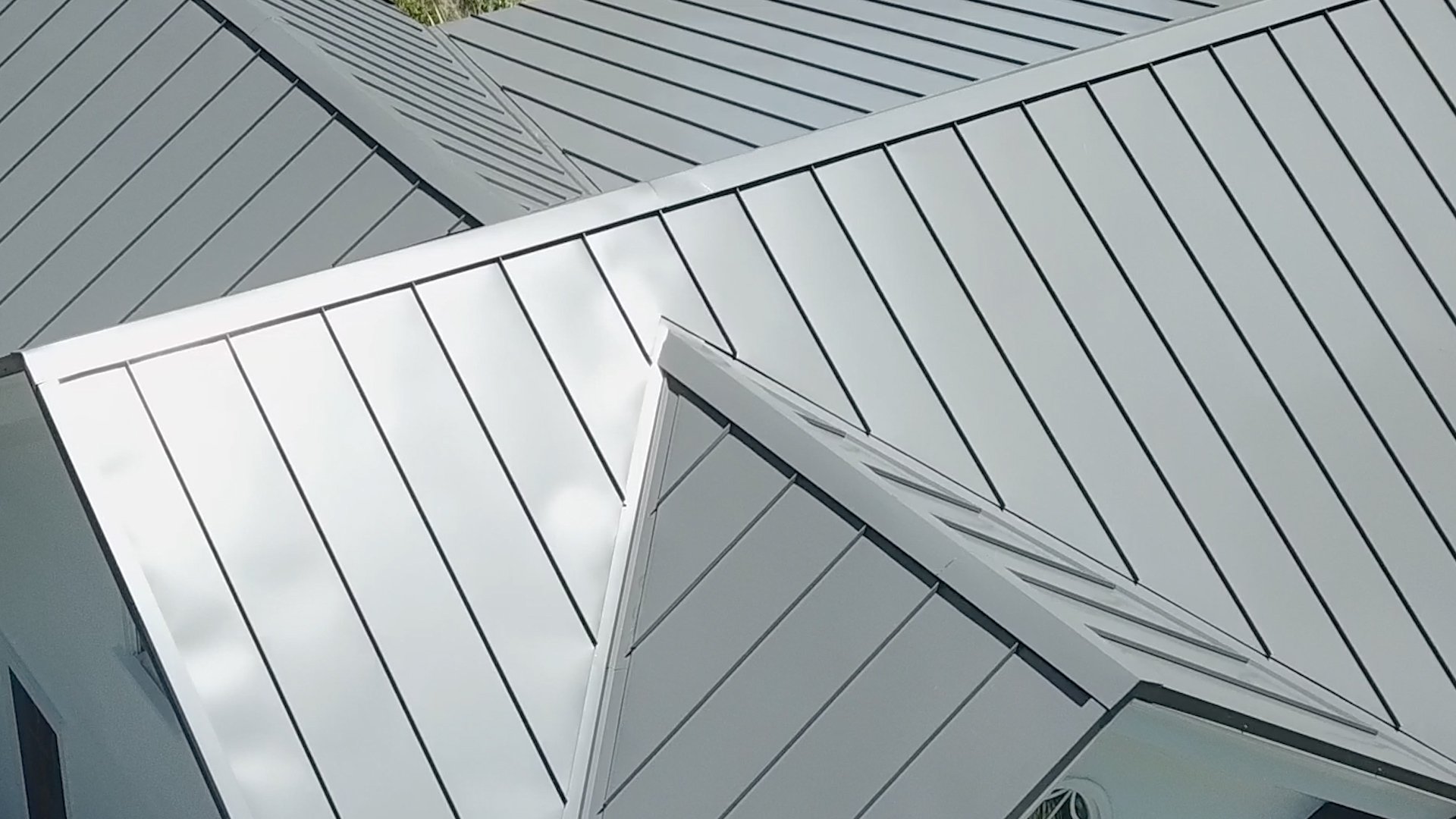The monochromatic image features a complex arrangement of a metal roof with multiple gables and dormers. The metal panels are arranged in vertical sections, joined at various angles, creating intricate geometric patterns. The central roof slopes diagonally from the upper right to the lower left of the image, forming a peak where several triangular and rectangular sheets converge. Below this, a flat rectangular section lies, connected to additional sheets that meet at complicated angles. The house’s white siding and windows are visible on the side, adding to the architectural details. A prominent dormer projects diagonally from the middle to the right side of the image, mirroring another dormer on the left side, while another gabled roof emerges from the back, maintaining the same panel pattern as the main roof.